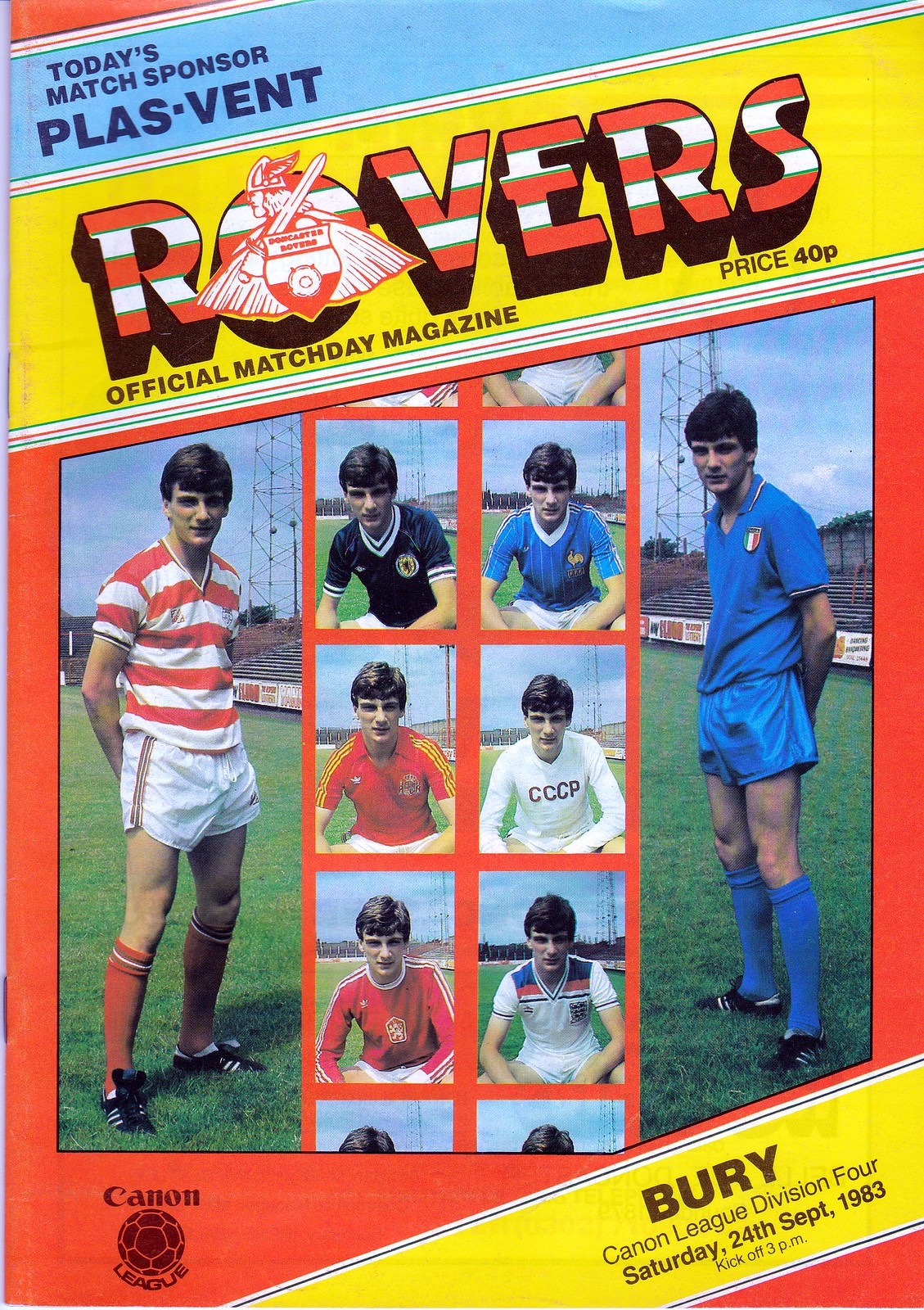The image is a vintage magazine cover from the 1970s or 1980s, showcasing "Today's Match Sponsor: Blast Vent" at the top against a blue background. Below this, in a yellow banner, is the title "Rovers," styled in red, white, and green. The cover features a logo depicting a knight with wings on his helmet, long hair, holding a sword, and wearing a cape. Under the logo, it reads "Official Match Day Magazine," priced at 40p.

Central to the cover are two photographs of the same gentleman. On the left side, he is wearing a red and white striped jersey, white shorts, red socks, and black cleats, standing in front of bleachers under a clear blue sky. On the right side, he appears in a blue uniform, from shirt to socks. Both images show him with a composed posture, hands clasped behind his back.

At the bottom, set against a yellow background, are the details of the match: "Bury Cannon League Division 4, Saturday 24th September 1983, kick-off 3pm." The worn look and the hairstyles suggest this is a piece of memorabilia from the 1970s or early 1980s.